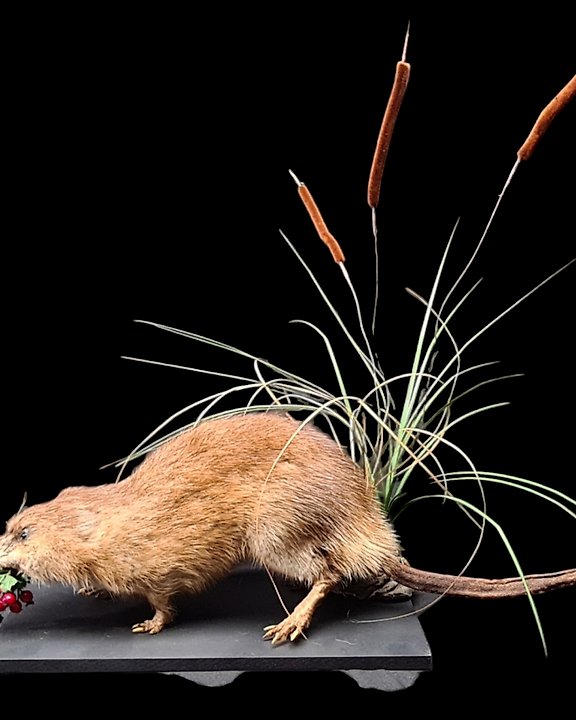The photograph showcases a taxidermied rat positioned on a black-painted metal shelf. The rodent, which appears to have beige fur, is clutching a bunch of cherries with leaves in its mouth. Its tail is partially cut off, and the remaining portion is brown. The rat sits in front of a green plant with thin leaves and fake sticks, all set against a black background. The rat’s eyes appear unfriendly, adding to its lifelike yet eerie presentation. Additionally, there are orange cylindrical elements, possibly flowers or pollen, mingling with the plant’s green foliage. Overall, the image focuses solely on the rat and the subtle details of its surroundings, emphasizing the artistry of the taxidermy.